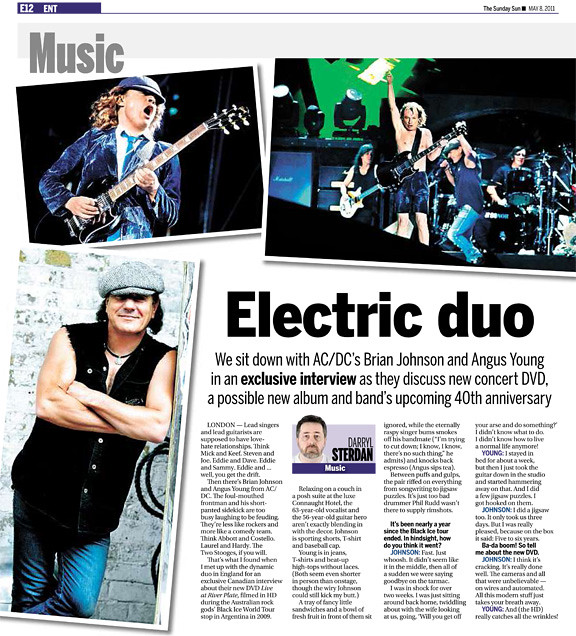The image depicts a page from the May 8th edition of the Sunday Sun magazine, specifically from the entertainment section, on page E12. The article is titled "Electric Duo" and features a detailed interview with ACDC’s Brian Johnson and Angus Young, as they discuss their new concert DVD, the possibility of a new album, and the band’s upcoming 40th anniversary. Written in London by music writer Daryl Sturden, whose headshot appears in the middle of the article, this piece is thoughtfully composed. The layout includes three photos: one on the left showing Brian Johnson standing against a wall in a sleeveless black shirt and jeans, another above it with Angus Young in his iconic schoolboy outfit playing guitar, and the third capturing the band performing energetically on stage.